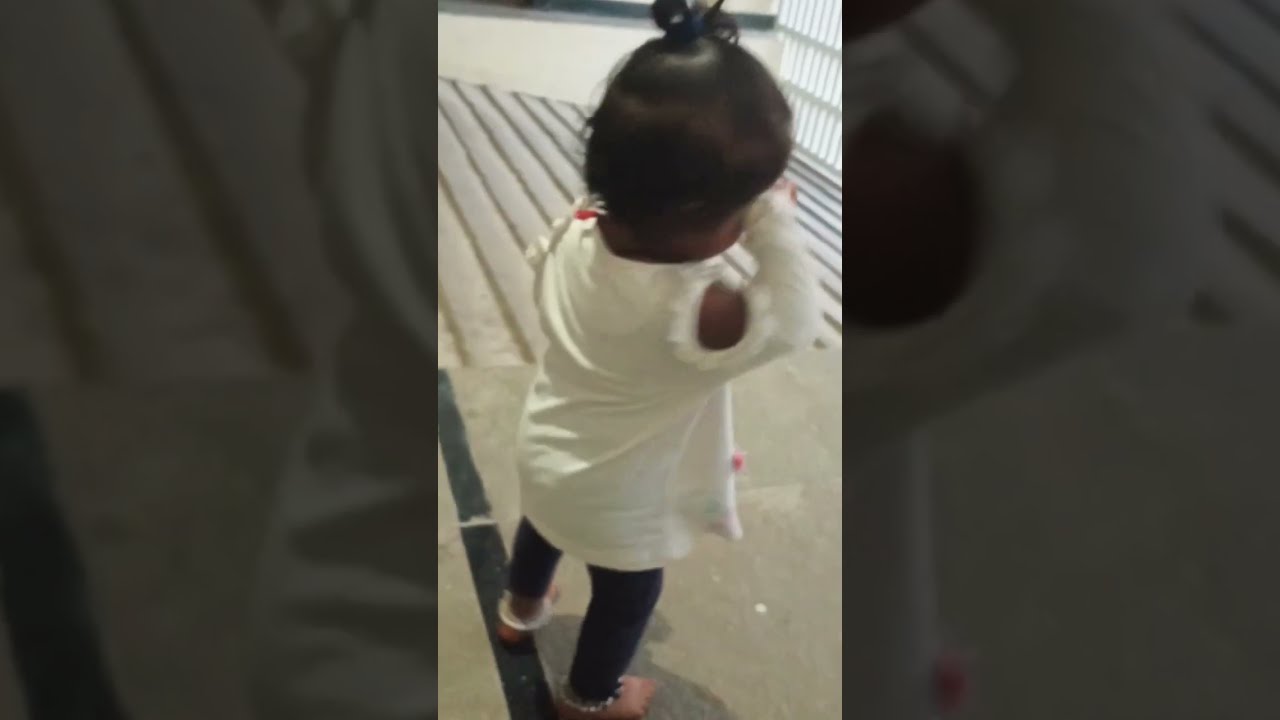In the center of the image, a photograph in portrait mode features a young child standing on the ground, facing away from the camera. The child’s dark hair is styled in a bun secured on top of her head, adorned with a small bow. She wears a white top with holes cut out on the shoulders, which are decorated with fake fur, and the shirt has pink buttons on the front. Additionally, the top has small decorative elements that resemble pink or red flowers or pom-poms. The child is dressed in dark leggings, either black or dark blue, and pink slippers with white fur around the ankles and pointed toes. The child has her hands raised to her face, suggesting she might be crying or rubbing her eyes. She stands on a surface made of white or grey marble tiles intersected by a strip of black concrete, with a white railing situated about ten feet away. Adjacent to this setting, a stair-like pathway is visible. The background of the entire image is filled with a blurred close-up of the main photograph, intensifying the focus on the young girl in the middle.